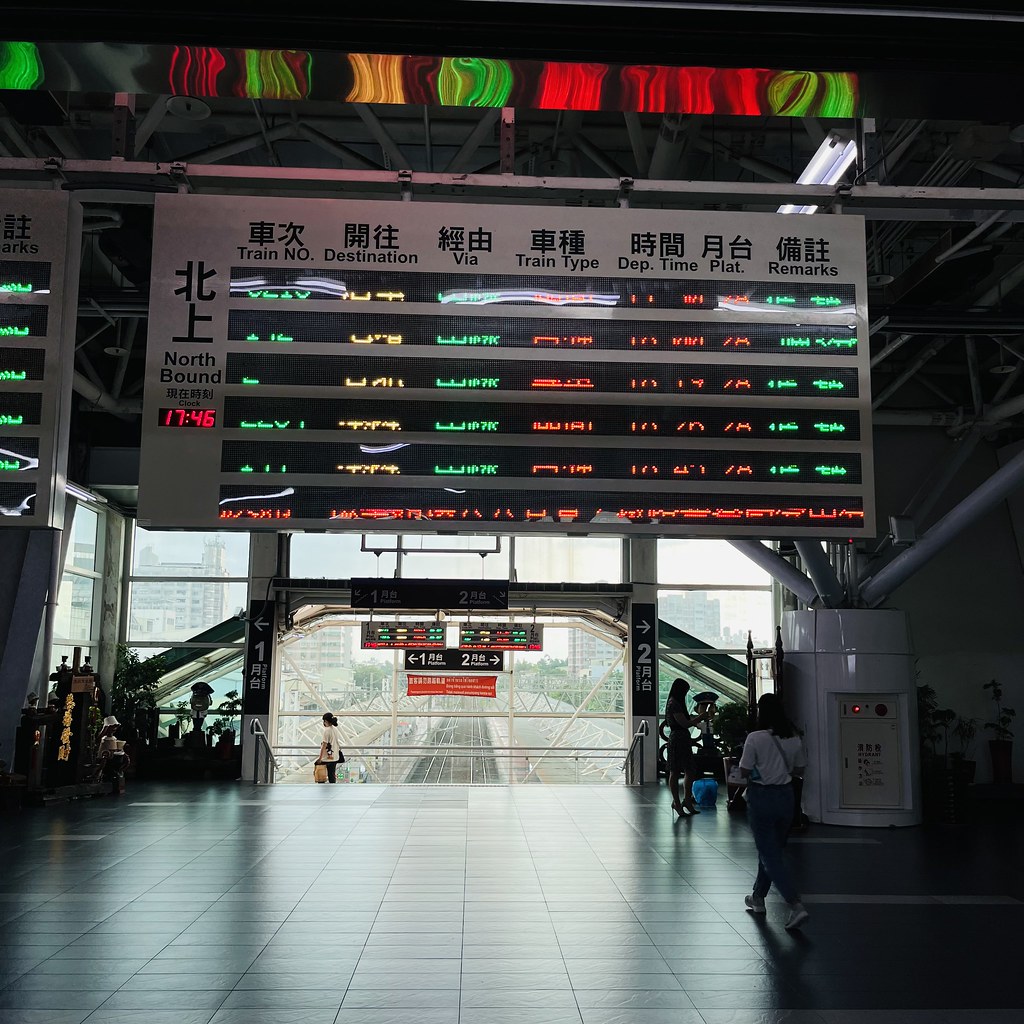The photograph captures the interior of an expansive train station, likely located in Asia, given the abundance of Asian characters present on signage. The bottom of the photograph reveals a large room culminating in a series of windows, through which train tracks and distant buildings are visible. 

A prominent feature at the top of the image is a large informational board with a silver outline on the left and top edges. The board contains multiple columns, each labeled with headings such as "Train Number," "Destination," "Via," "Train Type," "Departure Time," "Platform," and "Remarks." Below these headings, information is displayed in various colors including green, yellow, and orange. Additionally, there is a long black strip at the bottom of the board displaying information in orange text.

Several people are visible within the station. On the right side, one individual wearing a white shirt walks away from the camera. A couple of others can be seen in the distance; one facing right and another at the bottom of a short flight of stairs toward the middle left of the room. Furthermore, the right side of the room features a white kiosk and a bench positioned in front of it.

The overall scene is bright, especially towards the windows that allow natural light to stream into the station, creating a luminous atmosphere reminiscent of an airport terminal.